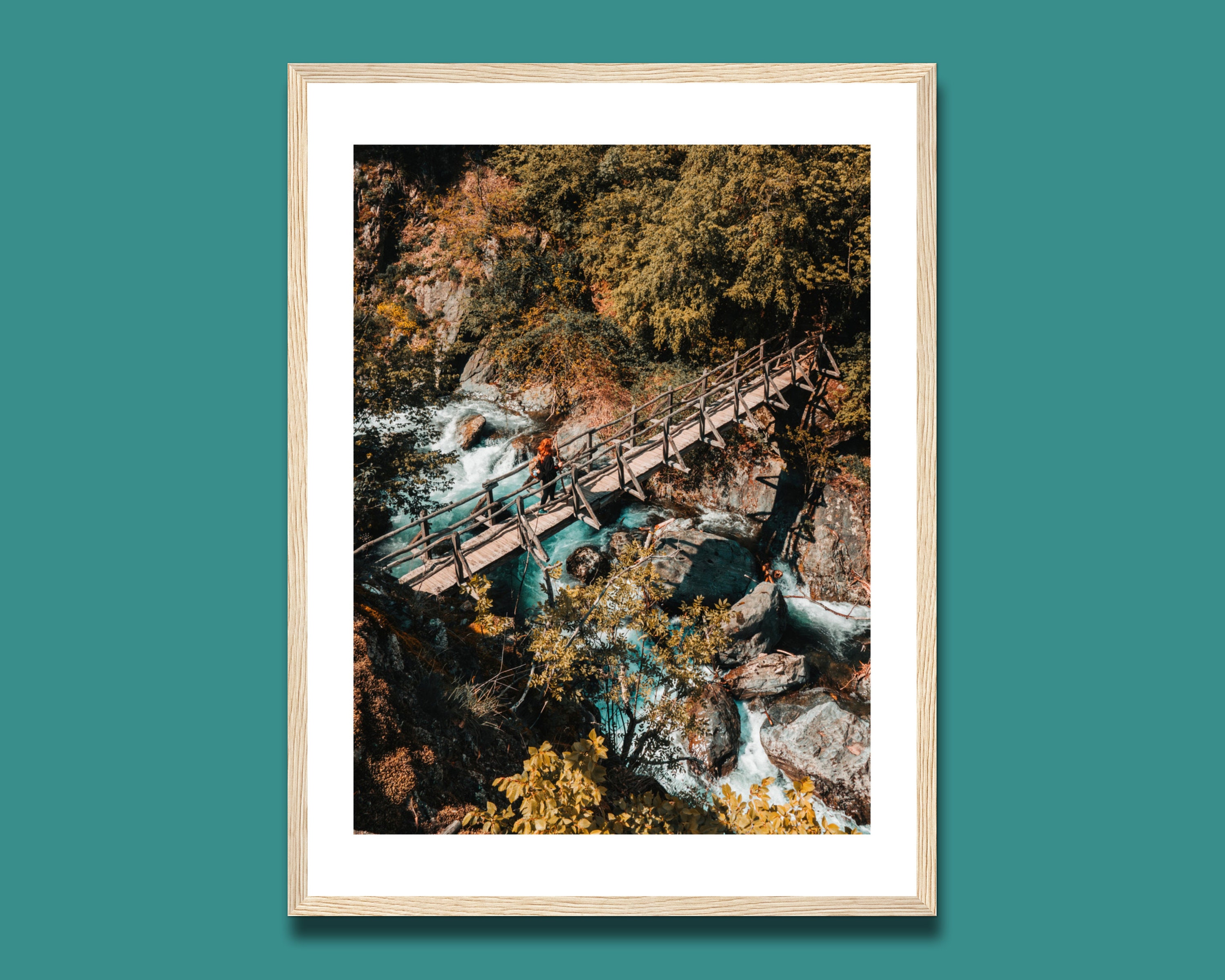This image features a framed photograph set against a mint green to teal blue background. The frame is gold, possibly metal, with a white border matting the picture inside. The photograph captures a serene landscape with a wooden bridge spanning a river or stream amidst a rocky terrain lined with both green and golden-hued trees. The water appears to be flowing swiftly around the large rock formations. At the center of the image, a person is halfway across the bridge, possibly wearing a hat or a red scarf, but their face remains obscured. The hillside ascends where the bridge connects, especially on the right side, while the left side of the image is slightly cut off at the bottom corner. The viewpoint appears to be aerial, providing a comprehensive yet slightly indistinct perspective on the natural scenery.